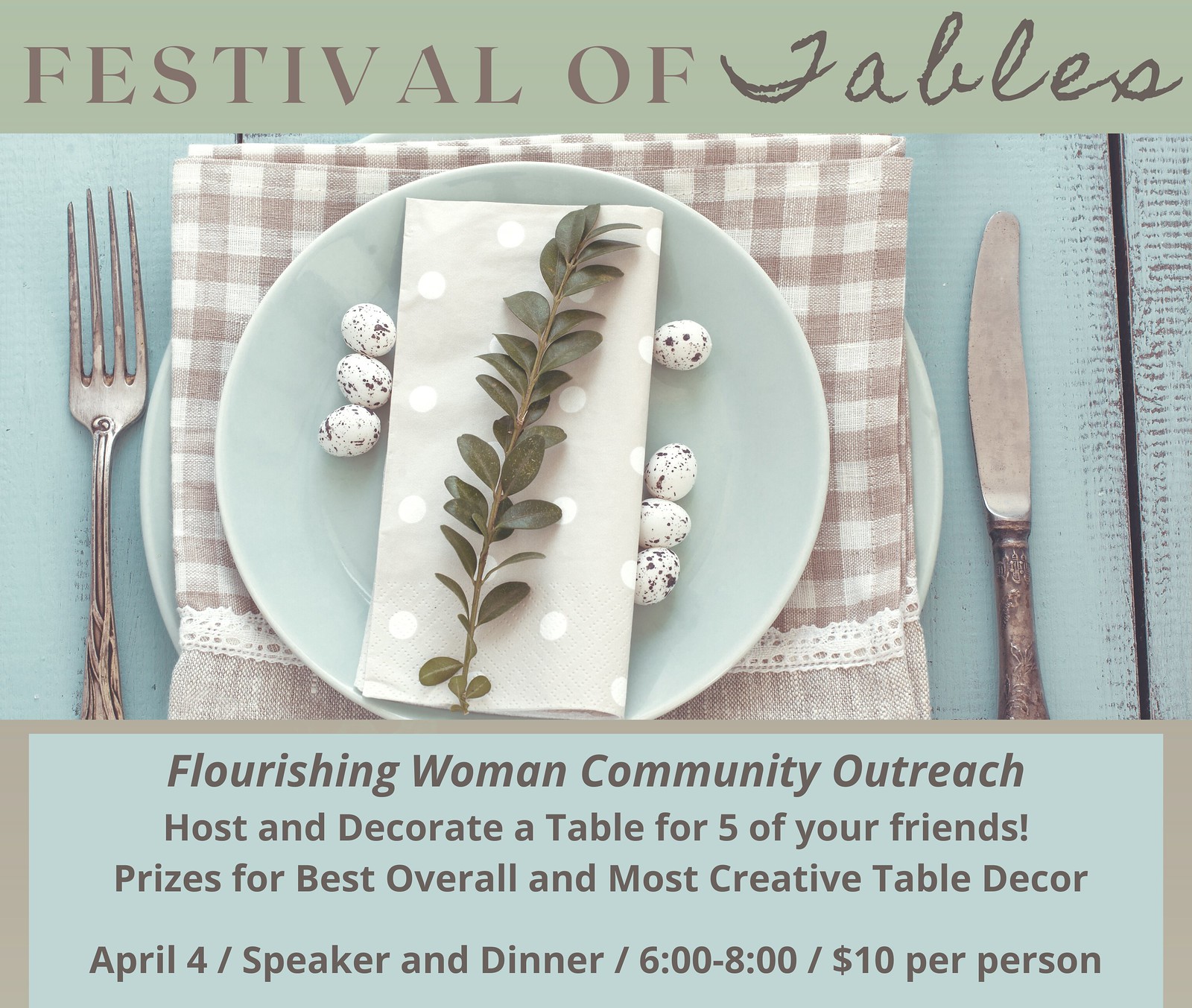Across the top of the graphic is a light green banner with the text "Festival of Fables" in a brown font. Below it, the words "The Lord of Fables" appear in a darker brown, handwritten style. Central to the image is a photo of an elegant table setting: a light blue plate holds a white, polka dot folded napkin adorned with a sprig of leaves. Surrounding the napkin are seven speckled eggs. The plate rests on a rustic brown and white checkerboard napkin, flanked by an antique silver fork and knife. The bottom part of the graphic features the text "Flourishing Women Community Outreach" in brown font, inviting the viewer to host and decorate a table for five friends. Additional details include prizes for the best overall and most creative table decor, with an event on April 4, featuring a speaker and dinner from 6-8 PM, priced at $10 per person.